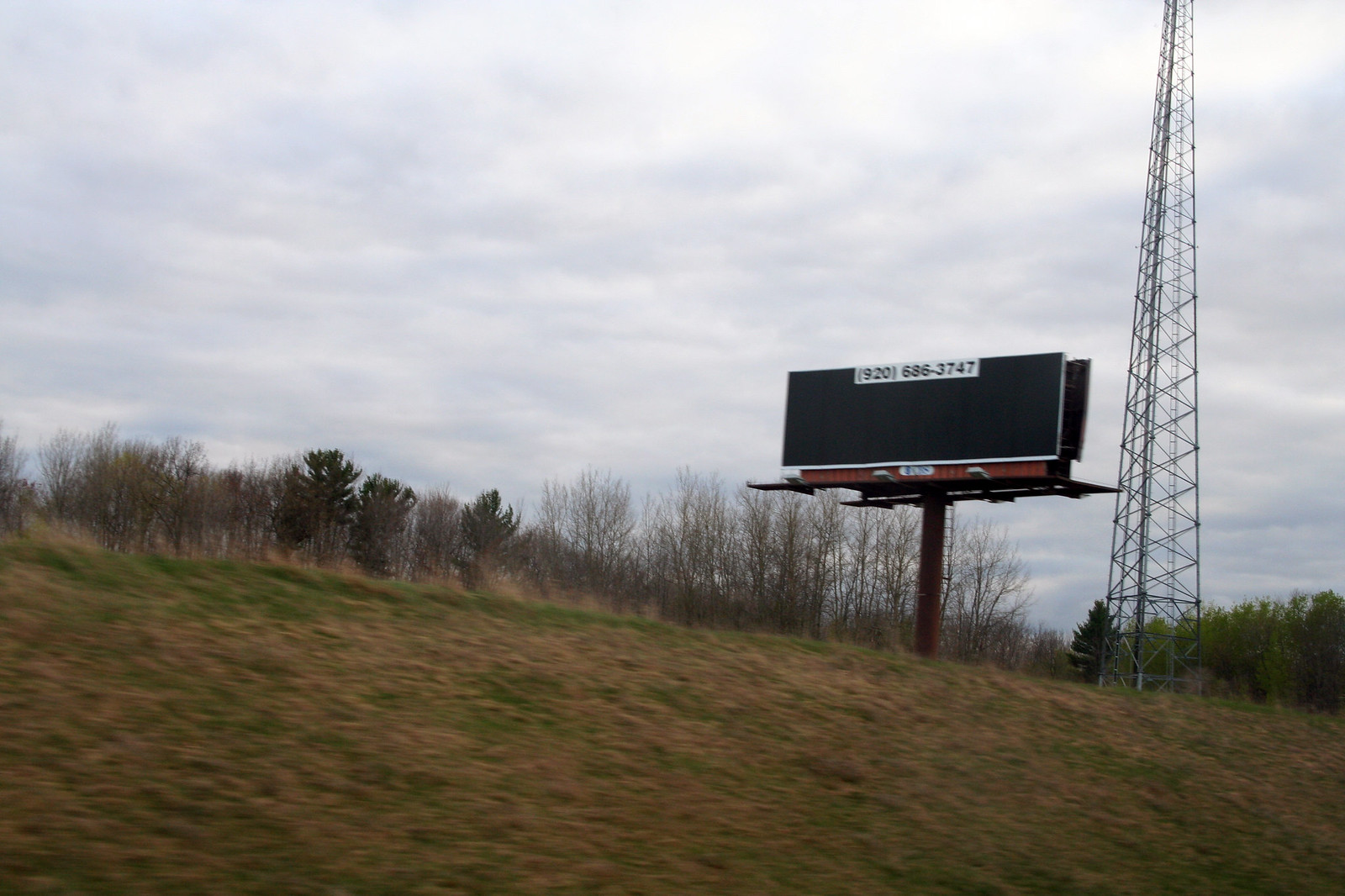The image captures a gently sloping hillside adorned with patches of green and brown grass. In the background stands a black billboard sign, currently unused, with visible contact information for future sign placements. Towering above the landscape, yet not fully visible in the frame, is a tall structure that appears to be a cell phone or radio tower. The sky overhead is dotted with clouds, while the silhouettes of trees, some shedding their leaves likely due to the onset of fall, frame the scene. On the right side, a tree line adds dimension to the landscape, with sparse vegetation and a few more trees populating the left side, creating a sense of natural balance and serenity.